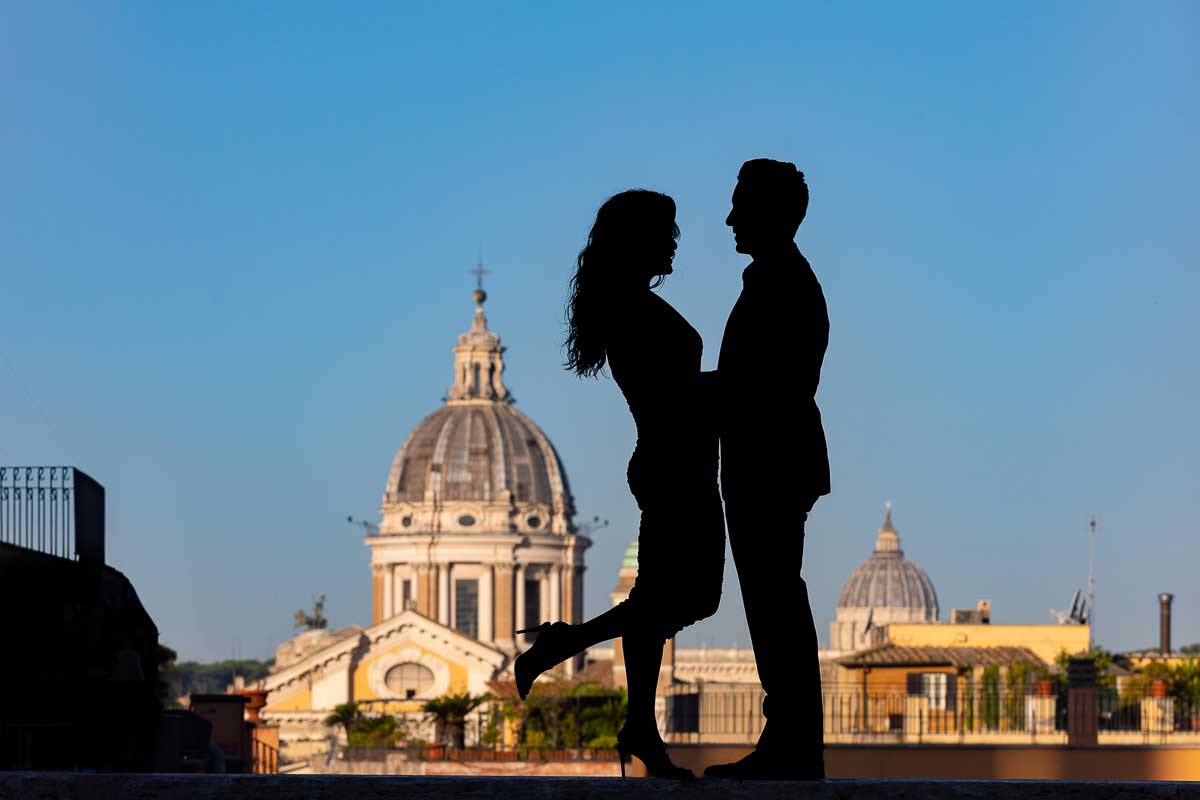In this striking image, a black silhouette of a couple stands in the foreground just right of center, against a background that could pass for a photograph. The woman, placed on the left, exudes grace with her long, wavy hair cascading down and her high-heeled right leg elegantly lifted behind her. She is petite in build, wearing a dress that falls just below her knee, with noticeable curves accentuated by her posture. Her arms are intertwined with those of the man to her right, who appears to be wearing a suit. Both figures are blackened shadows, providing no discernible details other than their outlines and postures.

The background reveals a picturesque scene of old architectural beauty bathed in clear blue skies. To the left of the woman, a building with a domed top capped with a cross punctuates the skyline. Further behind the man, in the distance, another domed building is visible. Closer to the foreground, a small building with a fence stands out, contributing to the sense of depth and the detailed setting. The lower camera angle adds an almost cinematic quality, enhancing the statuesque presence of the couple against the timeless backdrop.